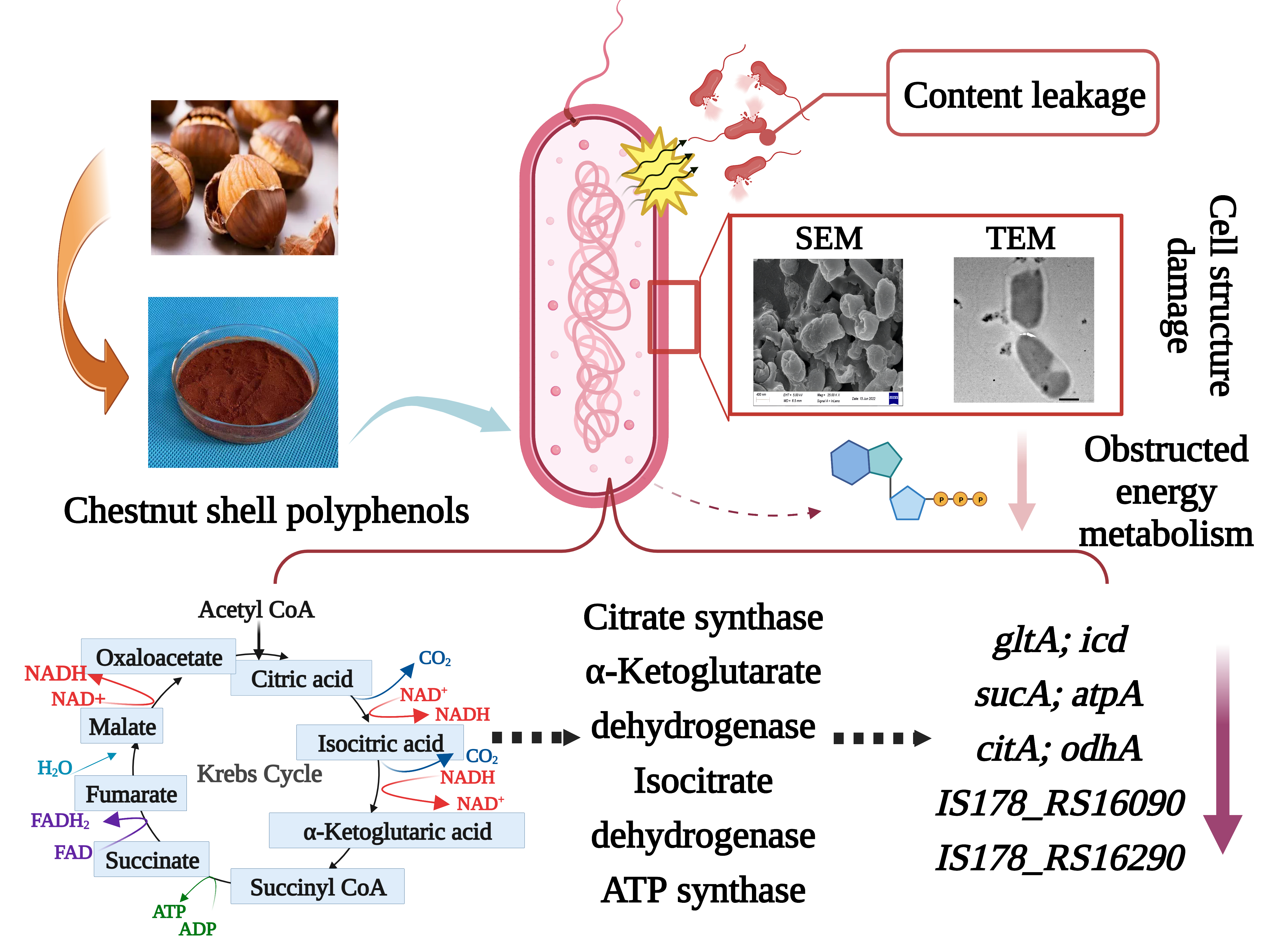The image is a detailed scientific diagram taken from a textbook about microscopic or cellular life, focusing on the processes affecting chestnut shells. In the upper left corner, there's a small photograph showing approximately five chestnuts. Beneath that is an image of a clear glass bowl containing a brown powder, labeled as chestnut shell polyphenols. To the right, a pink oval shape with intricate pink squiggly lines represents some chemical or cellular component, and it is connected to two black-and-white microscopic images labeled SEM and TEM. These images and the pink oval illustrate 'content leakage,' 'cell structure damage,' and 'obstructed energy metabolism,' which are processes and damage pathways explained in detail within the diagram. The bottom section features a complex map of related chemical reactions and processes, including the Krebs cycle, with numerous chemical names and symbols illustrating the metabolic and structural changes occurring to the chestnut shells. The purpose of the diagram is to provide a comprehensive explanation of what happens to chestnut shells at the microscopic level, highlighting the breakdown and the cellular impacts.